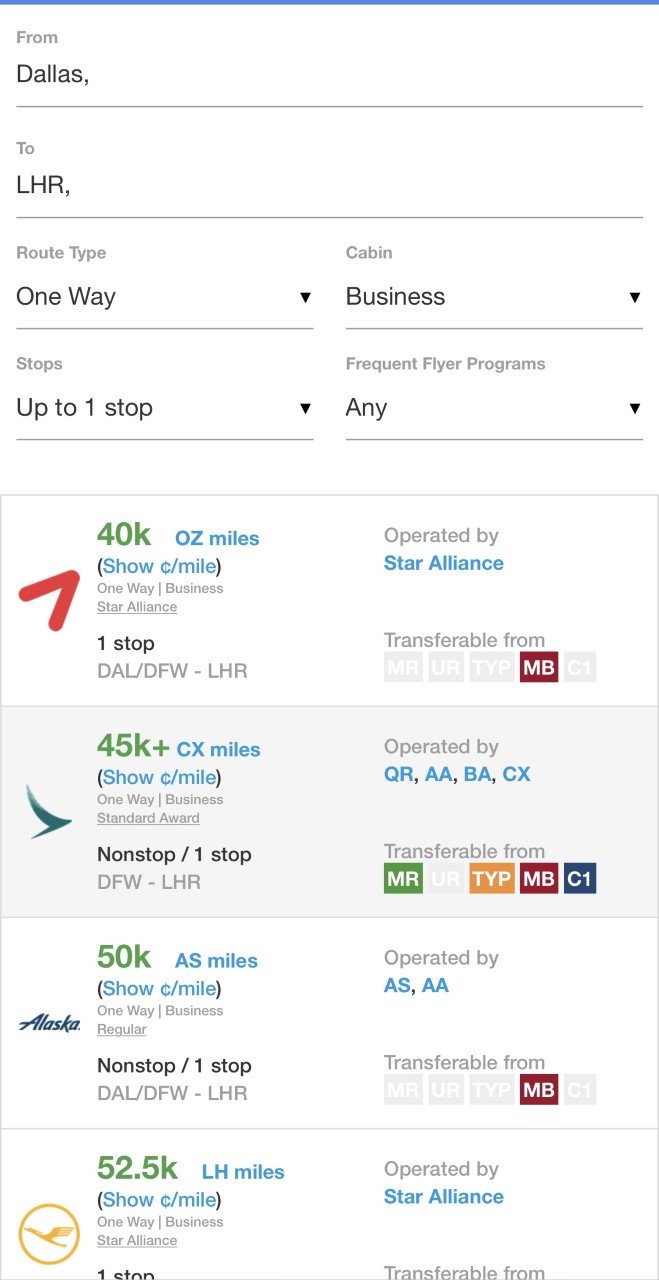Screenshot of a travel website displaying several flight options:
- **Form Details:**
  - Departure: Dallas (DFW)
  - Destination: London Heathrow (LHR)
  - Route Type: One-way
  - Cabin Type: Business Class
- **Flight Specifications:**
  - Stops: Up to one stop
  - Frequent Flyer Program: Any
- **Options Presented:**
  - First Set:
    - 40k OZ Miles
    - Show cents per mile
    - One-way Business
    - Star Alliance
    - One stop
    - Operated by Star Alliance
  - Second Set:
    - 45k plus CX Miles
    - Show cents per mile
    - One-way Business Standard Award
    - Non-stop
    - One-stop
    - DFW to LHR
    - Operated by QRAABACX
  - Third Set:
    - 50k AS Miles
  - Fourth Set:
    - 52.5k LH Miles